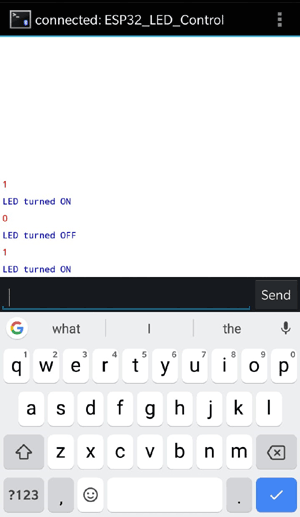The image is a screenshot with a predominantly white background. At the top, it displays a connection status message: "ESP32_led_control." Three vertical dots, which typically denote additional options, are visible. In the main section, there are indicators showing the states of LEDs: one is turned on, another is off, and a third is turned on again.

Below this section, there is a search bar with a visible cursor. Accompanying the search bar is a gray rectangle featuring sand and white colors. Within this rectangle, a white circle contains the letter "G" in Google's signature multi-color style, indicating the Google search symbol.

The keyboard interface appears at the bottom of the image. It includes lettered keys with numbers one through zero positioned on top of them. The keyboard also features an up arrow key, a key with a question mark, an "ABC" key, a key marked "123," a comma, a smiley face icon, the space bar, a period key, a key resembling a left-turned house with an 'X,' and a blue square highlighting a white check mark. Additionally, a microphone icon is visible, suggesting a voice input option.